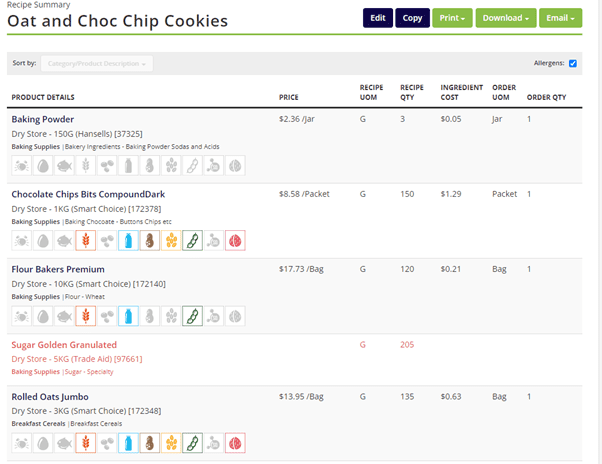This image showcases a recipe summary displayed on a digital device. At the top, in the upper-left corner, small print reads "Recipe Summary," while larger print below it lists the recipe title as "Oat and Chocolate Chip Cookies." Adjacent to the title, on the right, are various action buttons: a black "Edit" button, a black "Copy" button, and three green buttons labeled "Print," "Download," and "Email."

Beneath this row, there is a sorting option labeled "Sort by Category." The chosen category has a blue check mark next to "Allergens." Further down, under "Product Details," the image lists key ingredients: "Baking Powder," "Chocolate Chip Bits (Compound Dark)," "Flour (Baker's Premium)," "Sugar (Golden Granulated)," and "Rolled Oats (Jumbo)." Each ingredient entry includes colorful icons representing different categories and details about the item.

Additionally, beside each ingredient, the image shows related information such as the price, quality, ingredient cost, and order quantity, providing a comprehensive and organized summary for making Oat and Chocolate Chip Cookies.